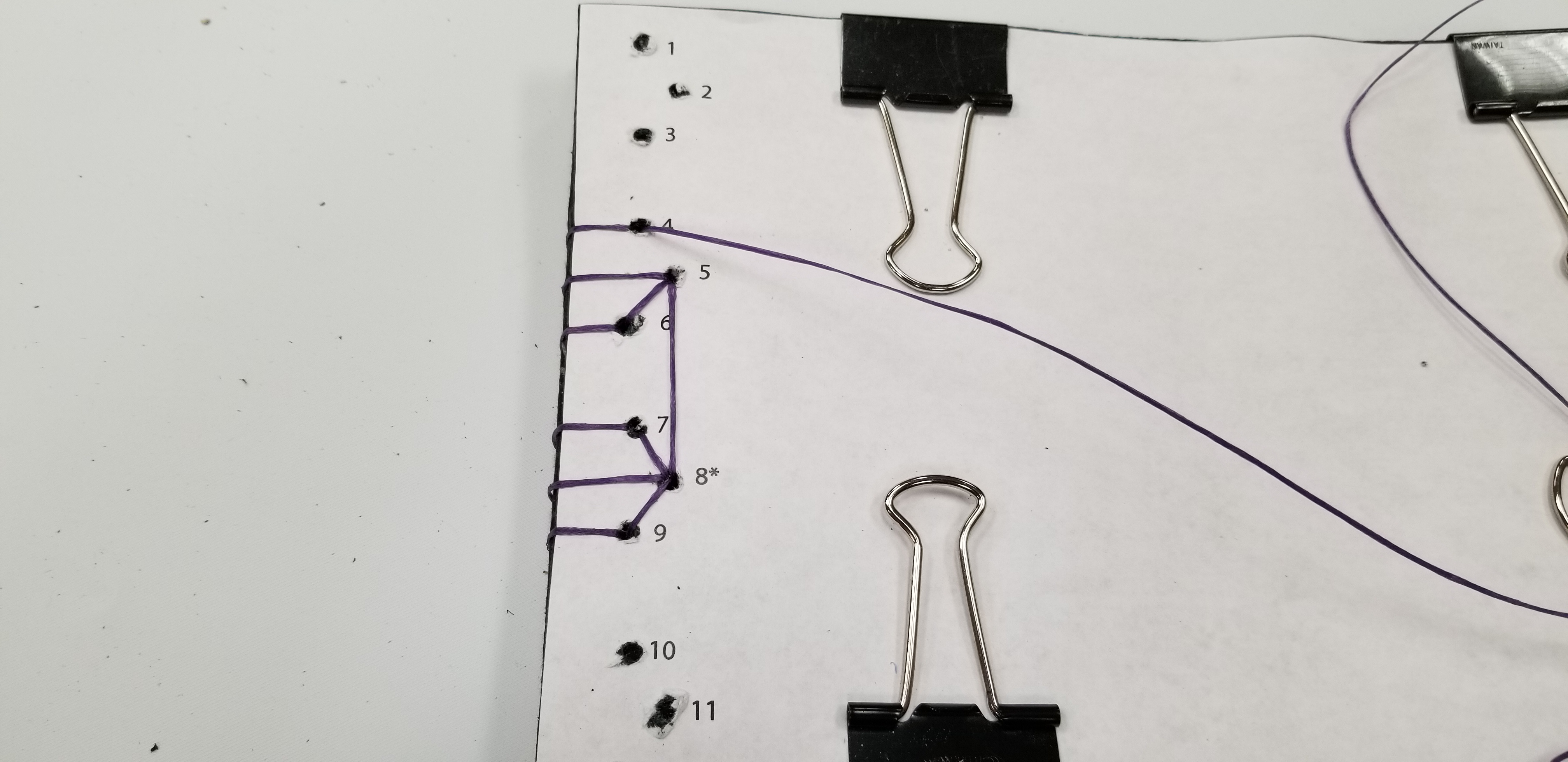This image features an open notebook lying flat on an undefined surface, with no discernible background. The notebook's inner seam, positioned slightly to the left of center, creates a darker line. The right page exhibits a series of evenly spaced, gray pencil-drawn dots that run parallel to the seam, just to its right. Approximately one-third from the top of the right page, a single black line arcs gently upward and then slopes downward, resembling a hill, before leveling off near the lower right corner. 

At the top of the notebook, two black metal binder clips, each with silver wire handles, are clipped to both the left and right sides, poised to secure the notebook's pages. Additionally, another black metal binder clip is positioned centrally at the bottom, just slightly off-center, mirroring the placement of the clip at the top left. This bottom clip is also fully extended with its wire brackets facing upward, ensuring the notebook remains spread open.